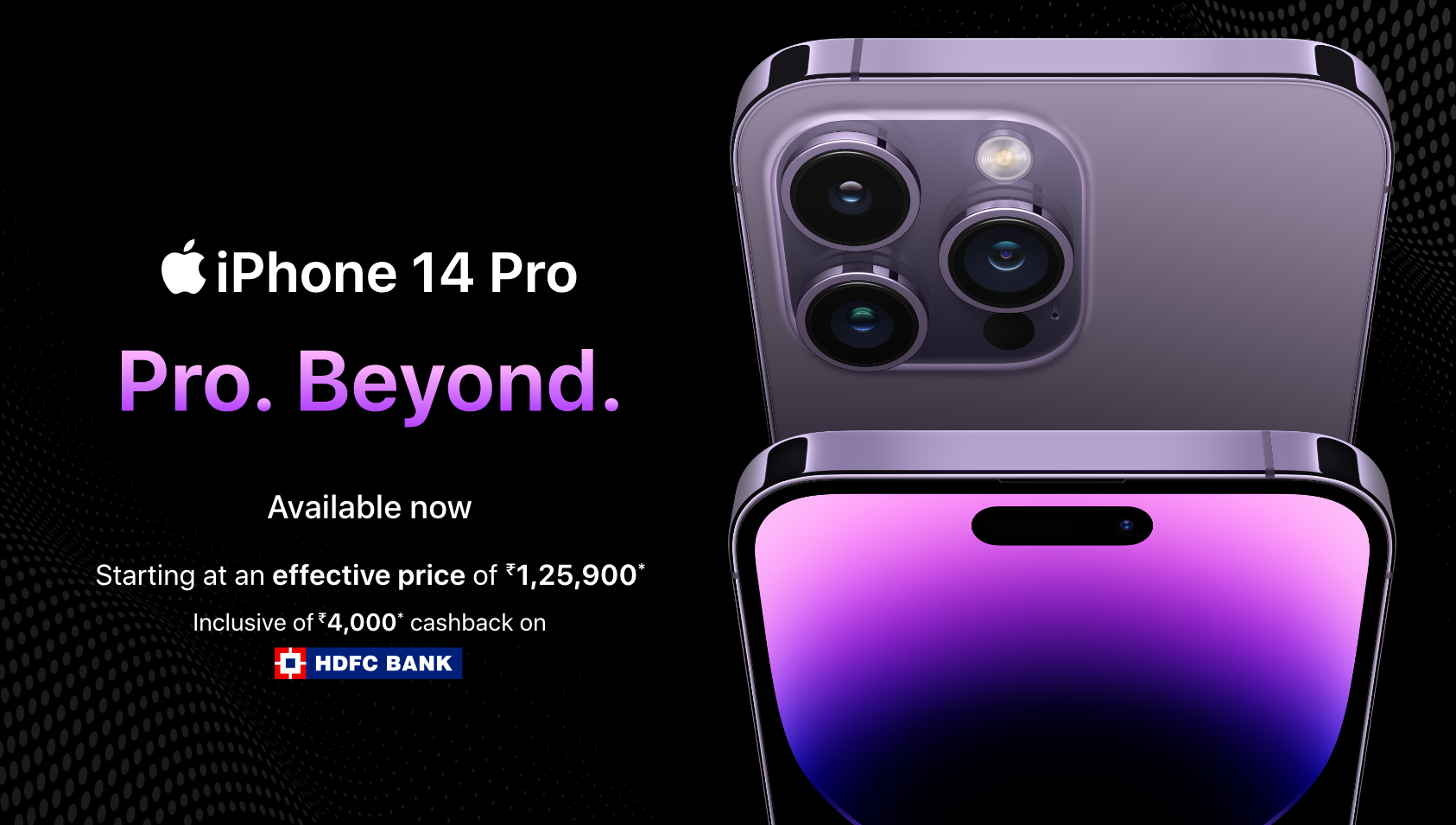Introducing the Apple iPhone 14 Pro! This sleek and elegant smartphone features a stunning purple finish, accented by highly reflective silver edges. Showcased prominently is the vibrant, colorful screen that sits below a trio of advanced cameras located at the top-right corner. 

The back of the phone highlights its model name, "Apple iPhone 14 Pro," along with the tagline, "Pro. Beyond." An attractive advertisement notes the mobile device starts at an impressive price point of $1,249.99, with enticing offers, including $4000 cash back on Blu-ray HD and HDSP purchases. 

The phone’s interface includes a visible button, enhancing its user-friendly design. Overall, this advertisement effectively captures the premium quality and advanced technology of the iPhone 14 Pro, presented in a refined purple hue.